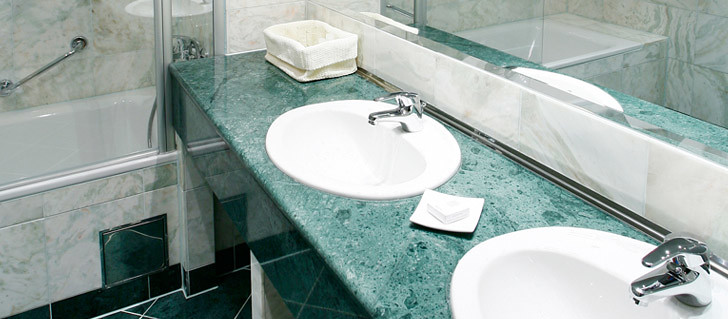This image captures the interior of a meticulously designed bathroom, showcasing a blend of elegance and modernity. Central to the photograph are two distinct sinks positioned side-by-side, set into a striking turquoise granite countertop that exudes sophistication. This vivid counter runs parallel to a sleek silver trim bar, which delineates the transition to the exquisite marble-tiled wall above. The marble tiles, with subtle hints of brown and gray, add a touch of luxury and texture to the space. 

A large, pristine mirror looms above the sinks, reflecting light and creating an illusion of spaciousness. On the countertop, a prominent square basket crafted from a cloth-like material sits empty, providing a touch of rustic charm. Between the sinks lies a neatly placed flat square soap dish, holding a pristine white bar of soap, emphasizing the bathroom's clean and organized ambiance.

The floor continues the turquoise theme with its matching tiles, grounding the room in a cohesive color scheme. To the left of the sinks, the marble tiles extend to the wall surrounding a versatile bath-shower combo. This unit features a practical silver grab bar for safety and convenience, complemented by a functional sliding glass door that enhances the shower's accessibility and modern appeal. The overall design harmonizes functionality with aesthetic finesse, making it a quintessential example of contemporary bathroom decor.